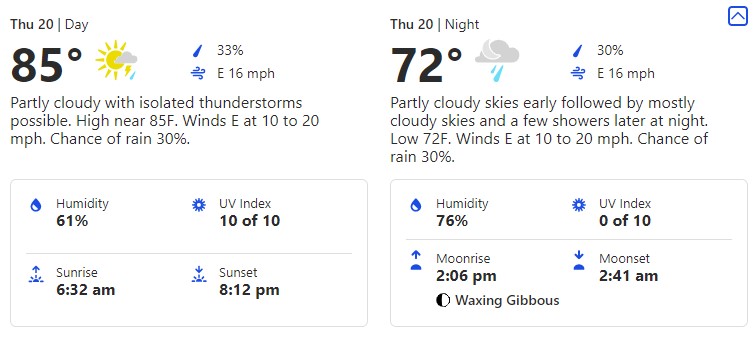Screenshot of a weather app display showing detailed forecasts for Thursday, the 20th. 

**Morning Forecast:**
- **Temperature:** 85°F
- **Wind:** Eastern winds at 16 mph
- **Humidity:** 61%
- **UV Index:** 10 out of 10
- **Sunrise:** 6:32 AM
- **Sunset:** 8:12 PM
- **Conditions:** Partially cloudy with a possibility of isolated thunderstorms, high near 85°F. Winds east at 10-20 mph, with a 30% chance of rain.
- **Icons:** Sun partially obscured by a cloud, with a raindrop indicating possible rain.

**Night Forecast:**
- **Temperature:** 72°F
- **Wind:** East winds at 16 mph
- **Humidity:** 76%
- **UV Index:** 0 out of 10
- **Moonrise:** 2:06 PM
- **Moonset:** 2:41 AM
- **Lunar Phase:** Waxing gibbous
- **Conditions:** 30% chance of rain.
- **Icons:** Cloud with a moon and two raindrops indicating possible rain at night.

The forecasts present a clear distinction between day and night weather conditions with specific meteorological data, helpful notes about potential rain, and visual icons for easy interpretation.